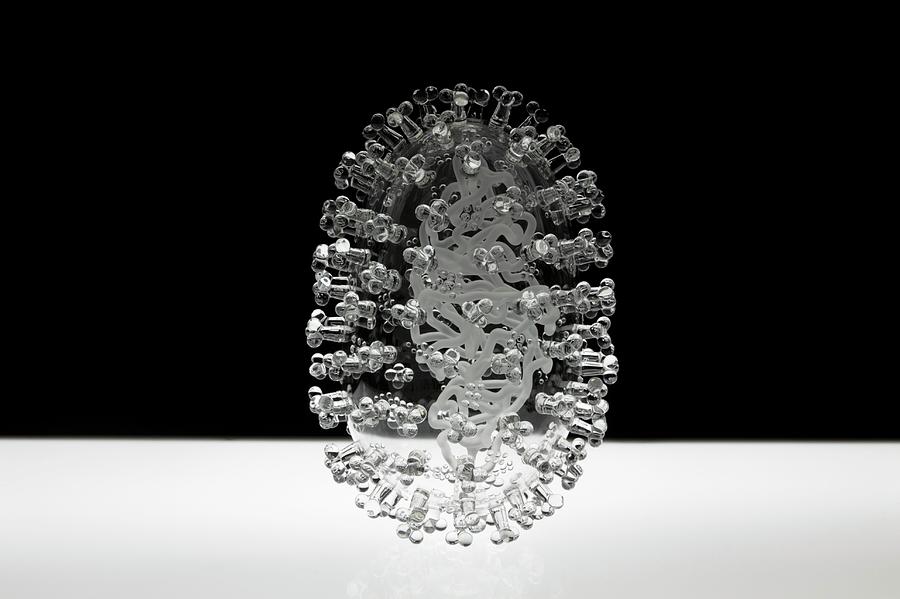This close-up image captures an abstract, oval-shaped structure that appears to be crafted from transparent or crystal-like material. The shape is adorned with numerous protrusions resembling glass or plastic knobs that encircle the outer edge and extend outward. The background behind the object is predominantly black (around 70%), seamlessly transitioning into a white section (approximately 30%), providing a stark yet soft contrast that highlights the structure's intricacies.

Inside the oval, interwoven, squiggly transparent lines crisscross in a pattern reminiscent of an intricate tapeworm or the convoluted structure of the human brain. These internal lines suggest a complex, organic form and add depth to the clear outer shell. The background seen through the object shifts in tone, making the protrusions appear gray against the black and almost clear against the white. This play of light and shadow gives the structure an ethereal and delicate appearance, emphasizing its abstract, mechanical beauty. The overall effect is a stunning, almost microscopic view of a crystal-like form that melds the organic with the geometric.